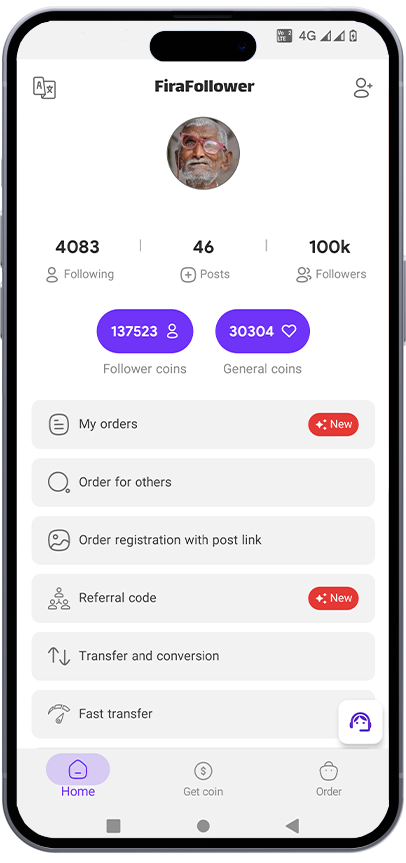The image showcases a smartphone screen displaying the Fira Follower app interface. The phone's status bar at the top indicates a 4G connection and battery life icons. The app's name, "Fira Follower," is prominently displayed with "Fira" and "Follower" both starting with capital letters.

Central to the screen is a circular avatar of a man who seems to be of Indian descent. He has short-cropped gray hair, a matching gray mustache, and beard, and wears red-framed glasses that sit at an angle on his face. Below the avatar, the user's statistics are listed: 4,083 people followed, 46 posts made, 100,000 followers, 137,523 follower coins, and 30,303 general coins.

Several options and sections are displayed beneath these statistics: "My Orders," "New," "Order for Others," "Order Registration with Post Link," "Referral Code," "New," "Transfer and Conversion," and "Fast Transfer." To the right of these options is a square white icon depicting a person wearing a telephone headset, often symbolizing customer support.

The bottom navigation bar of the app shows three icons: "Home" (which is currently selected), "Get Coin," and "Order."

Overall, the image is portrait-oriented (taller than it is wide) and contains no images of animals, birds, plants, flowers, trees, or automobiles.